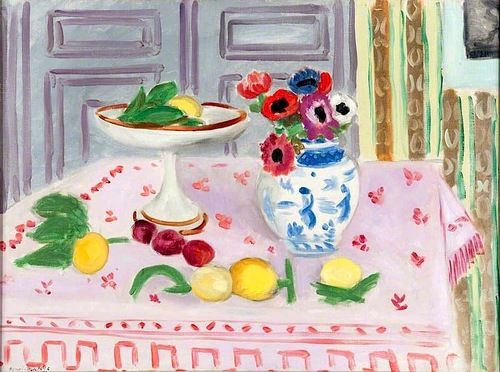This detailed painting captures a still life scene, focusing on a table adorned with a pink and white tablecloth featuring delicate red leaf patterns and a decorative frill. The table is laden with a variety of fruits including lemons, possible oranges, and potentially apples or cherries, as well as some leafy greens. Centrally placed on the table is a distinctive white fruit bowl with brown trim, elevated on a pedestal, holding additional green fruits or vegetables and a yellow fruit. 

A prominent blue and white Delft-style vase stands to the side, brimming with a vibrant arrangement of flowers in shades of red, orange, purple, white, and blue, including pansies. In the background, the scene is set against purplish-gray double doors and wallpaper with a yellow and brown pattern. To the right of the table, vertical brown signs with white lettering appear, potentially spelling out "H-O-H-A." The overall composition is rich in color and texture, drawing attention to the ornate details and the lush assortment of still life elements.